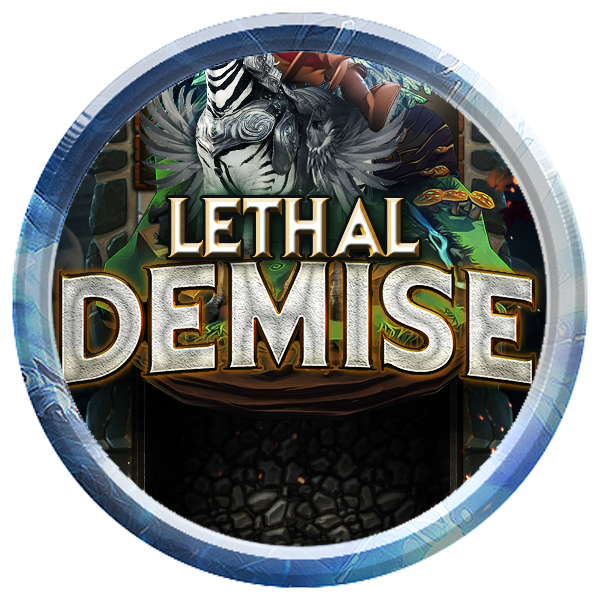The image depicts a highly stylized graphic design focusing on a large, circular emblem centered against a plain white background. The emblem features a textured, beveled outer ring blending various shades of blue and white, reminiscent of icy hues. This ring encircles the core of the design, which prominently displays the text "Lethal Demise" in the center. The word "Lethal" appears in beveled white text, while "Demise" is rendered in a metallic silver, enhanced with a black outline and an additional orange outline.

Inside the circular emblem, there is a detailed scene: at the top, a zebra adorned with gray armor and feathers stands on a vibrant green patch of land, dotted with small orange mushrooms. Below this, at the bottom of the scene, different types of stones and a dark textured wall or road are visible. The surrounding elements, including hints of a stream and granary, contribute to the depth and complexity of the illustration. The overall style suggests it could be a logo or design associated with a game or cartoon, evoking a fantastical and adventurous aesthetic.